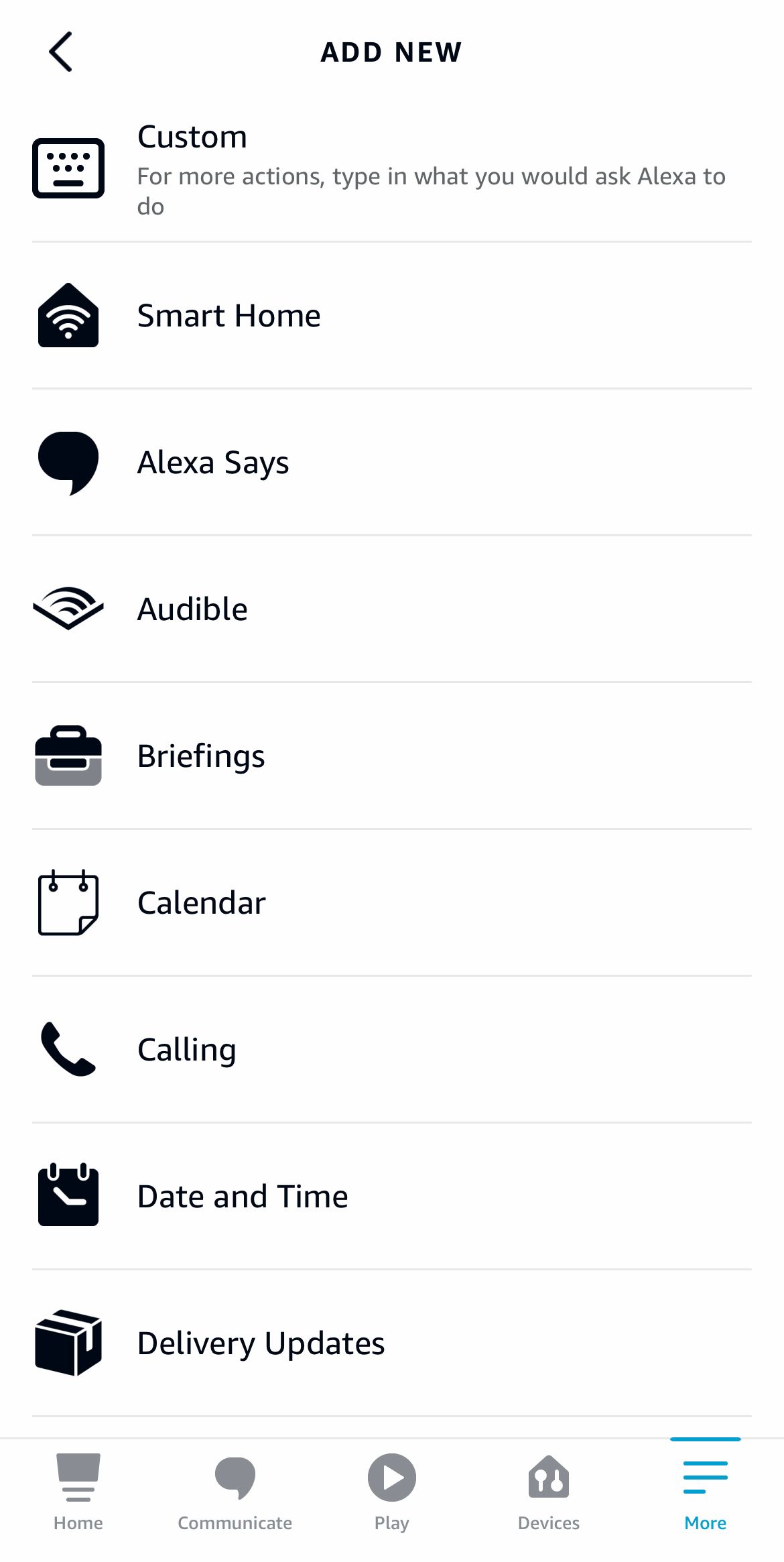This black and white screenshot, taken from a mobile or tablet device, showcases the "Add New" section of an Amazon Alexa setup. The image has been carefully cropped to exclude any web browser details or the physical device itself, focusing solely on the interface. Below the "Add New" title, a list of action items is neatly displayed, each accompanied by a distinctive icon on the left. The items include "Custom," "Smart Home," "Alexa Says," "Audible," "Briefings," "Calendar," "Calling," "Date and Time," and "Delivery Updates." At the very bottom of the screen, a navigation bar features five logos, permitting the user to select between Home, Communicate, Play, Devices, and More. The "More" option is highlighted in blue, indicating the current selection. This visually minimalistic layout clearly belongs to an Amazon Alexa setup, designed to allow users to add and customize various actions for their Alexa device.